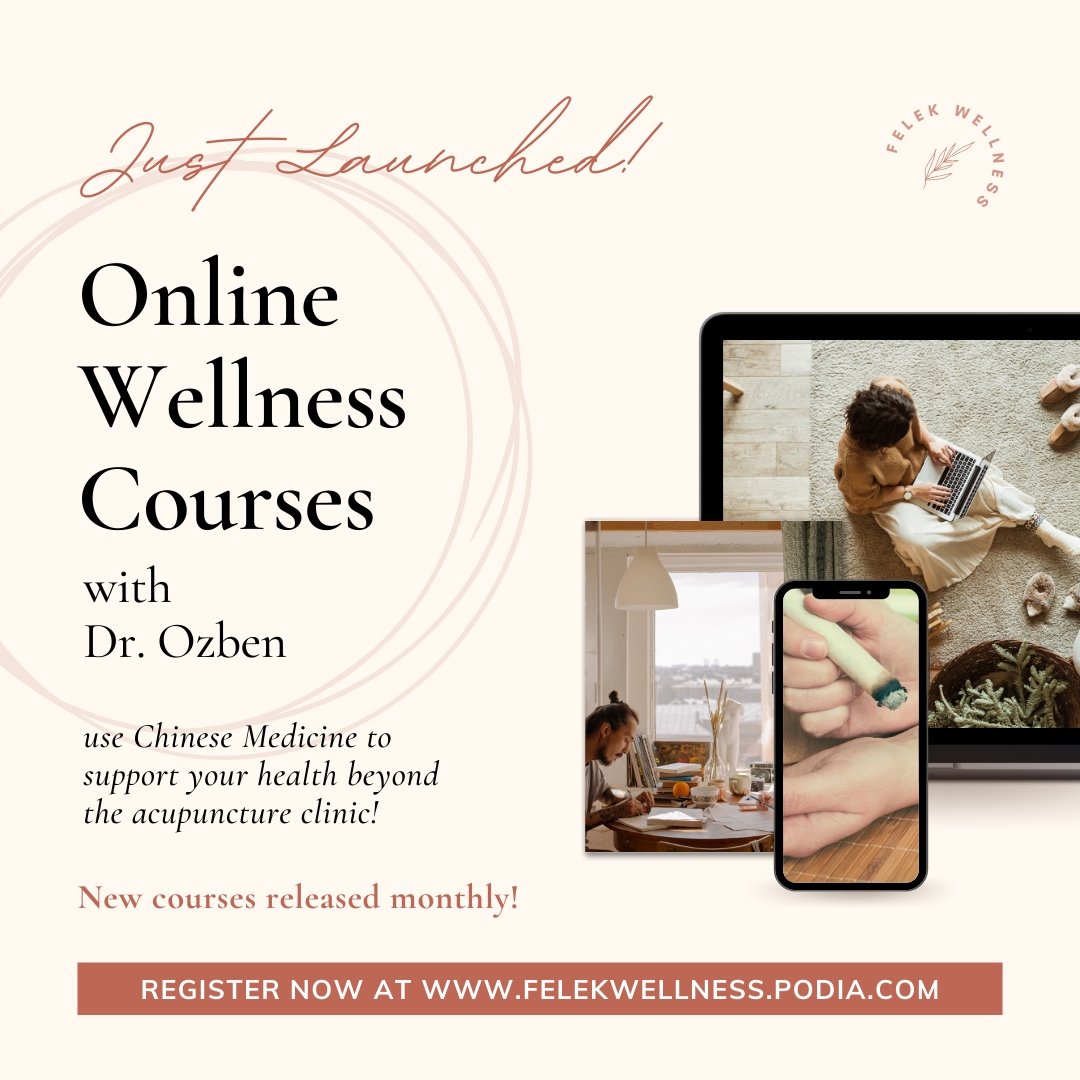### Detailed Caption for Online Wellness Course Website

The website for the newly launched online wellness courses features a visually appealing design with a pink-to-white gradient background. At the top, elegant script reads "Just Launched!" with the phrase "Online Wellness Course" in bold black letters directly below. Encircling this text is a hand-drawn pair of circles, adding a personal touch. The presenter of the course, Dr. Osbyn, is introduced within this graphic.

Positioned on the left side of the webpage, a compelling tagline reads, "Use Chinese Medicine to support your health beyond the acupuncture clinic!" in an eye-catching font. Directly beneath this, in pink text, another notable feature states, "New courses released monthly."

On the right-hand side, a striking visual component complements the text. A photograph showcases a tablet and a smartphone screen, where the tablet screen depicts a woman diligently working on a laptop. Adjacent to her image, on the left, is a detailed scene featuring an Asian man with a man-bun, seated at a table in his apartment, which offers a glimpse of the outdoors through a window. He appears focused and engaged in his work. Meanwhile, the smartphone screen displays a close-up image of two hands holding some form of smoking incense, adding an element of traditional wellness practices.

At the bottom of the page, a rust-colored rectangular box provides a call to action, stating, "Register now at www.flekwellness.podia.com." This section ensures that visitors know exactly where to sign up for the courses.